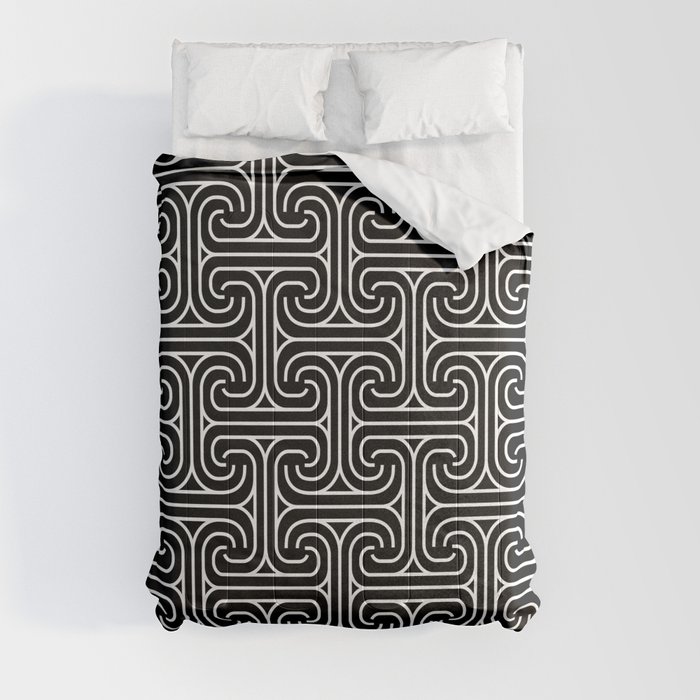This image depicts a square, six-inch by six-inch frame with a light bluish-gray background. At the center, there's a bed viewed from above. The bed, roughly four inches high and two to three inches wide, features a white sheet and two white pillows at the head. The bed is predominantly covered by a comforter that exhibits a unique, intricate pattern. This comforter is black with white geometric designs resembling curved capital 'I's or elongated 'C's nested within each other, running both horizontally and vertically, giving it a quilty texture. The top right corner of the comforter is slightly turned down, revealing its white underside, as though inviting someone to slip into bed. A darker shadow to the left of the bed provides some contrast against the light background.